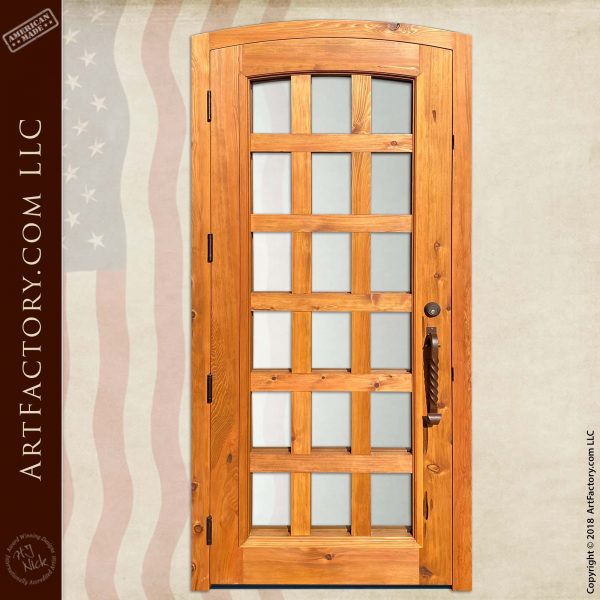The image showcases a close-up of a finely crafted wooden door, most likely a front or interior door. The door features a transparent United States flag superimposed over it, with the flag’s blue field and white stars, along with red and white stripes visibly integrated into the design. On the left side of the image, a black banner runs vertically, bearing the text "ArtFactory.com, LLC" and a brown mark along the left side also containing this text. At the top left corner, the phrase "American Made" is inscribed. The door itself is detailed with elaborate craftsmanship, consisting of a middle panel that includes 18 small glass window panes arranged in a 3x6 grid. Complementing this design are a metal handle and a lock mechanism on the right side of the door (left side from the viewer's perspective). Additionally, there is a copyright notice "© 2018, ArtFactory.com, LLC" positioned on the bottom right-hand corner, running vertically in black font. The door is mounted with four visible hinges on the left-hand side. There is also a circular logo towards the bottom that appears to say "H. J. Nick."